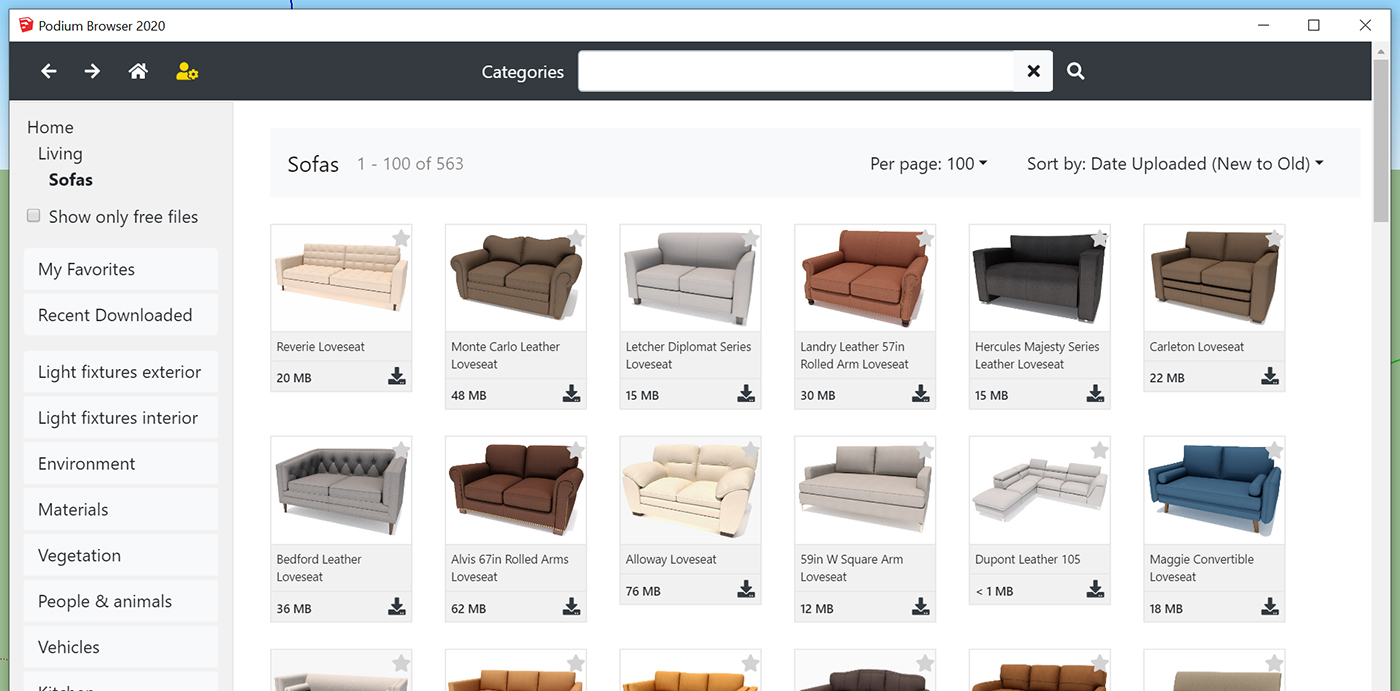The image showcases a webpage from the Podium Browser in 2020. In the top left corner, there's a distinct red and white icon followed by the text "Podium Browser 2020" in black. Spanning across the top of the page is a black bar featuring navigational icons: a left-pointing arrow, a right-pointing arrow, a home icon, and an icon of a person with a yellow circle around the right shoulder area. Centrally located within the bar is the text "Categories" in white, accompanied by a white search bar and a magnifying glass icon to its right.

On the left side of the page runs a vertical menu with various categories listed in black text. These include: Home, Living, Sofas, Showing Only Free Files, My Favorites, Recent Downloaded, Light Fixtures Exterior, Light Fixtures Interior, Environment, Materials, Vegetation, People & Animals, and Vehicles.

To the right of this menu section is the main content area. At the top left of this section, it reads "Sofas 1 to 100 of 563" with a dropdown menu labeled "per page, 100." Nearby, there's another dropdown for sorting options with the default set to "Sort By Date Uploaded (New to Old)."

The primary portion of the page is divided into rows displaying images of sofas and loveseats. There are two complete rows, each featuring six images. At the bottom, a partial third row is visible with the tops of six additional images, though it is truncated by the lower edge of the image.